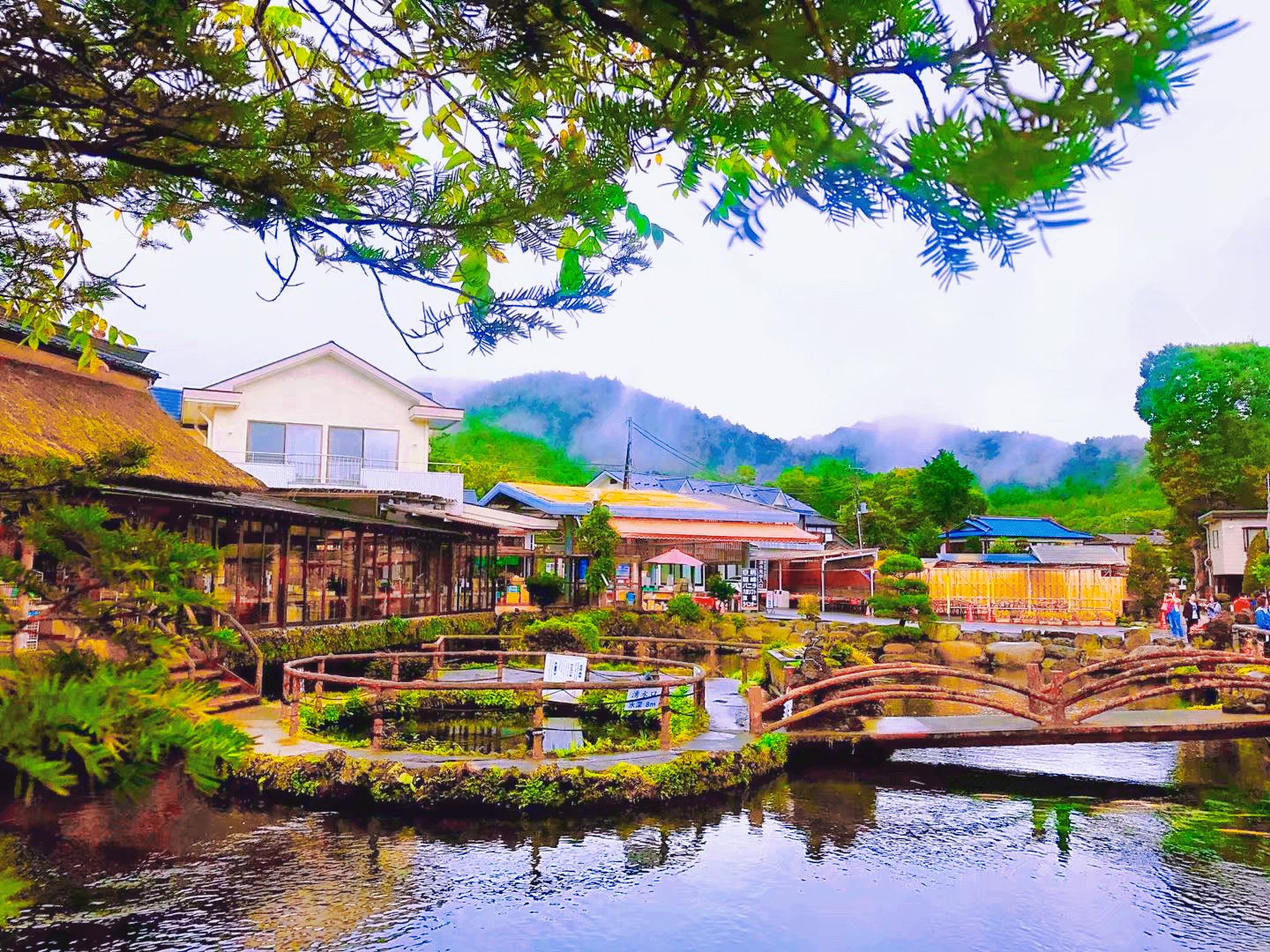This painting depicts a vibrant, picturesque village that’s nestled alongside a serene body of water. The scene has an ambiguous quality that makes it difficult to determine whether it's a painting or a photograph due to its semi-clear, detailed yet slightly indistinct rendering. At the forefront of the painting is a reflective lake, around which several colorful structures—likely businesses and homes—stand with varying tones of brown, white, yellow, and blue. A quaint bridge spans the lake, connecting to a small circular area that serves as an intersection for pathways. The background showcases a breathtaking view of mountains shrouded in fog or smoke with abundant, lush trees scattered throughout. A large tree branch stretches nearly across the top of the painting, with beams of sunlight filtering through, enhancing the richness of the greenery. On the far right, a few indistinct figures are barely recognizable near a large green tree. The village exudes a captivating charm with its multi-hued buildings, green forestry, and hints of daily life, suggesting it might be a serene yet lively shopping center by the lake.